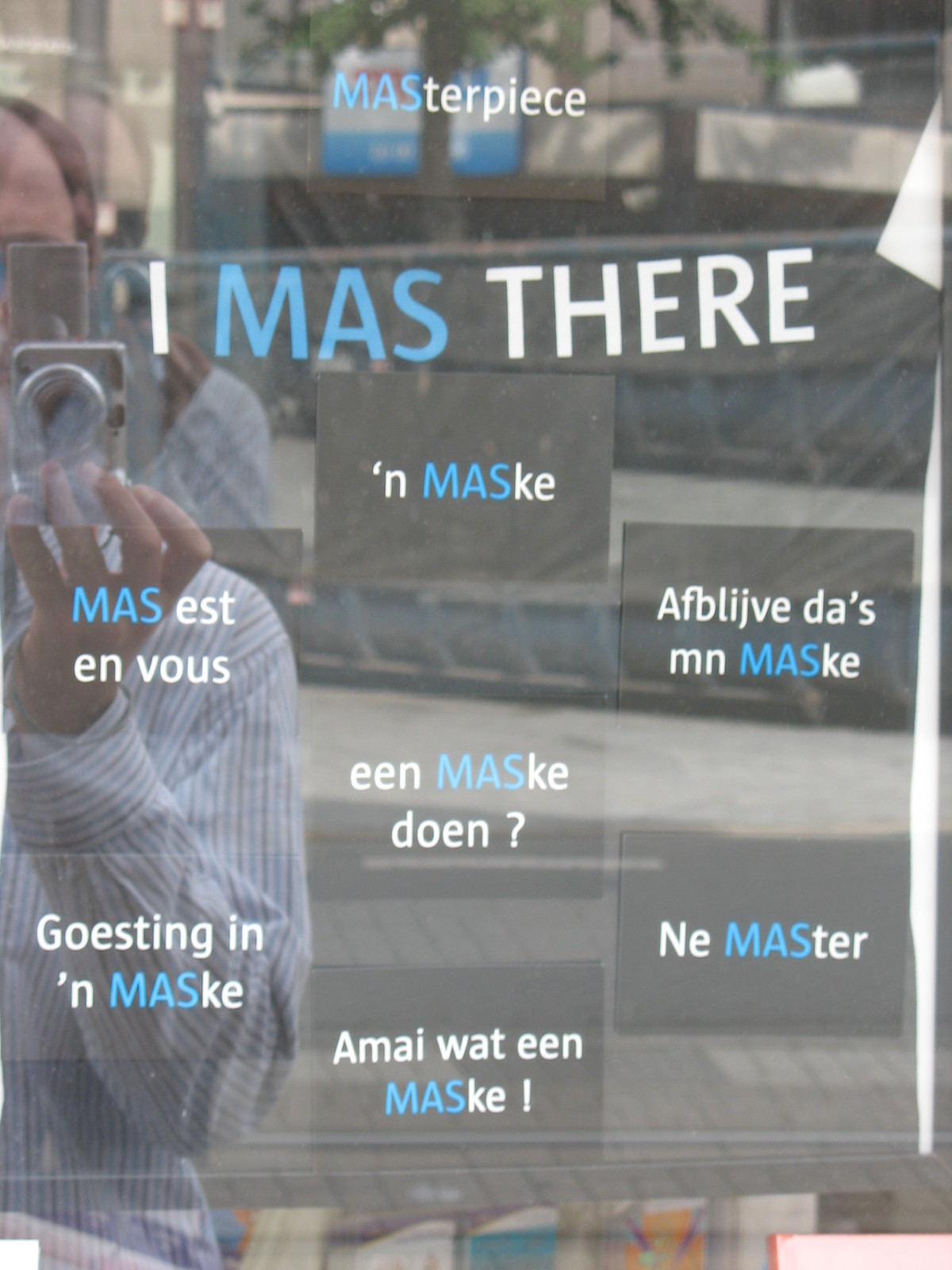The image is a vertically-oriented photograph of a window display, showcasing a series of cards with text written in a foreign language. The text includes phrases such as "I was there," "masterpiece," and "mas etant vous," where the words are printed in various colors like white and blue. The scene captures the slightly reflective glass of the window, revealing the reflection of the photographer, who is holding a camera vertically and wearing a white shirt with colored stripes.

To the left side of the image, partially cut off, is a man, likely the photographer himself. He appears to be slightly bald and is standing on a bridge. In the background, several stores, signs, and trees can be seen, indicating an outdoor setting in the middle of the day. The colors in the image range from gray, white, and light blue to black, orange, purple, yellow, and green, adding to the vibrant ambiance of the scene. Overall, the image focuses more on the textual elements rather than any particular object, creating an intriguing visual blend of reflections, language, and outdoor details.